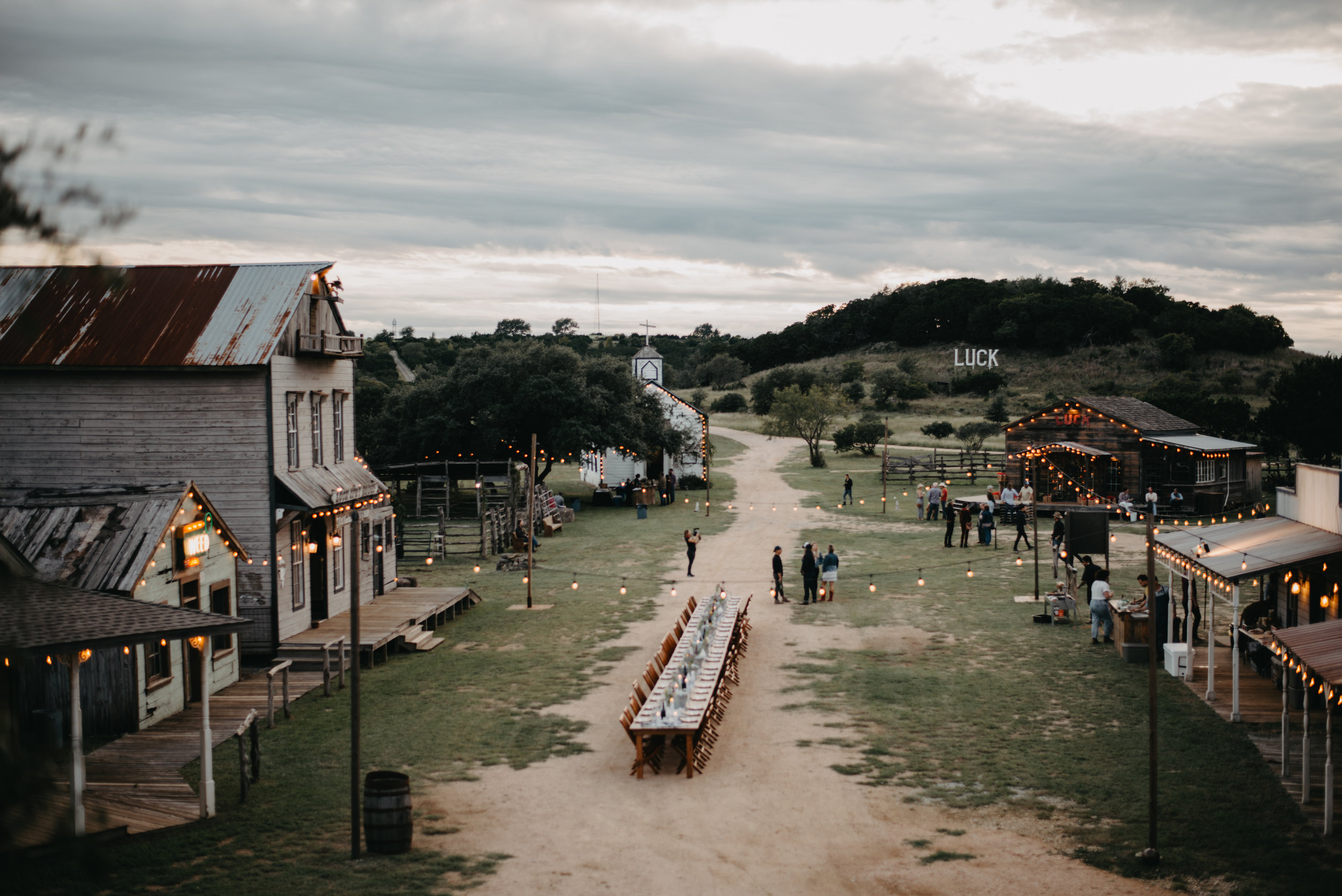The photo depicts a beautifully decorated, old-timey town that evokes the charm of the Old West, yet has a modern festive flair. Centered along a dirt road is a long table meticulously set up, likely for a grand reception or a celebratory dinner, complete with chairs and centerpieces. Strands of porch-style lights are strung between various older buildings and on the front porches, casting a warm glow that hints at evening time. People are seen milling around, adding to the lively atmosphere that suggests a party or a special event is in full swing. To the left, there are two buildings adorned with lights, while to the right, smaller houses also draped with Christmas lights further brighten the scene. In the background stands an all-white church, adding a serene touch to the festive ambiance. A wooden walkway, barrels, old light poles, and a neon sign contribute to the blend of historic and lively décor. Overlooking this picturesque setting is a small hill featuring a sign with the word "luck" on it. The sky is clouded and devoid of sunlight, suggesting it is the darkening hours of the evening.